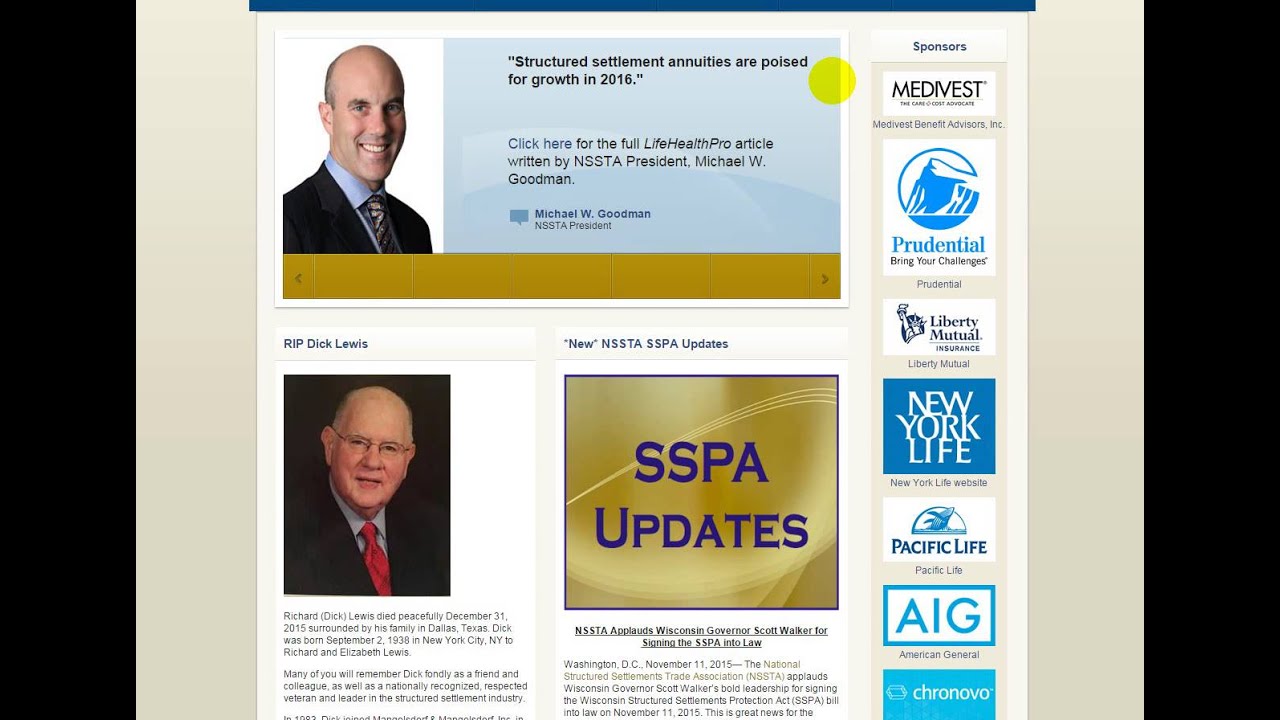This screenshot depicts a news webpage, potentially sourced from a news website. The top of the page features a prominent advertisement with the headline "Structured Settlement Annuities are Poised for Growth in 2018," indicating its nature as a promotional banner. 

Below the banner ad lies the core news story segment titled "SSP Updates." On the left, there is an image of an older man, likely in his 60s, attired in a black suit with a red tie. This image accompanies the text of the main news story. To the immediate right of this section, there's another related story under the "SSP Updates" header, showcased on a gold background with blue lettering.

Adjacent to the news story, on the far right-hand side of the webpage, there is a column filled with various advertisements for insurance companies, including Prudential, Liberty Mutual, New York Life, Pacific Life, and AIG, labeled as sponsors.

At the very top right corner, another advertisement features a younger man, approximately in his 30s to early 40s, inviting users to click for more information on structured settlement annuities, which are predicted to grow in 2018.

Overall, the webpage is considerably laden with advertisements, more so than a typical news page, with multiple insurance-related ads bordering the main content. The structured layout signifies the webpage's intent to provide news while simultaneously promoting related financial products through various ads.